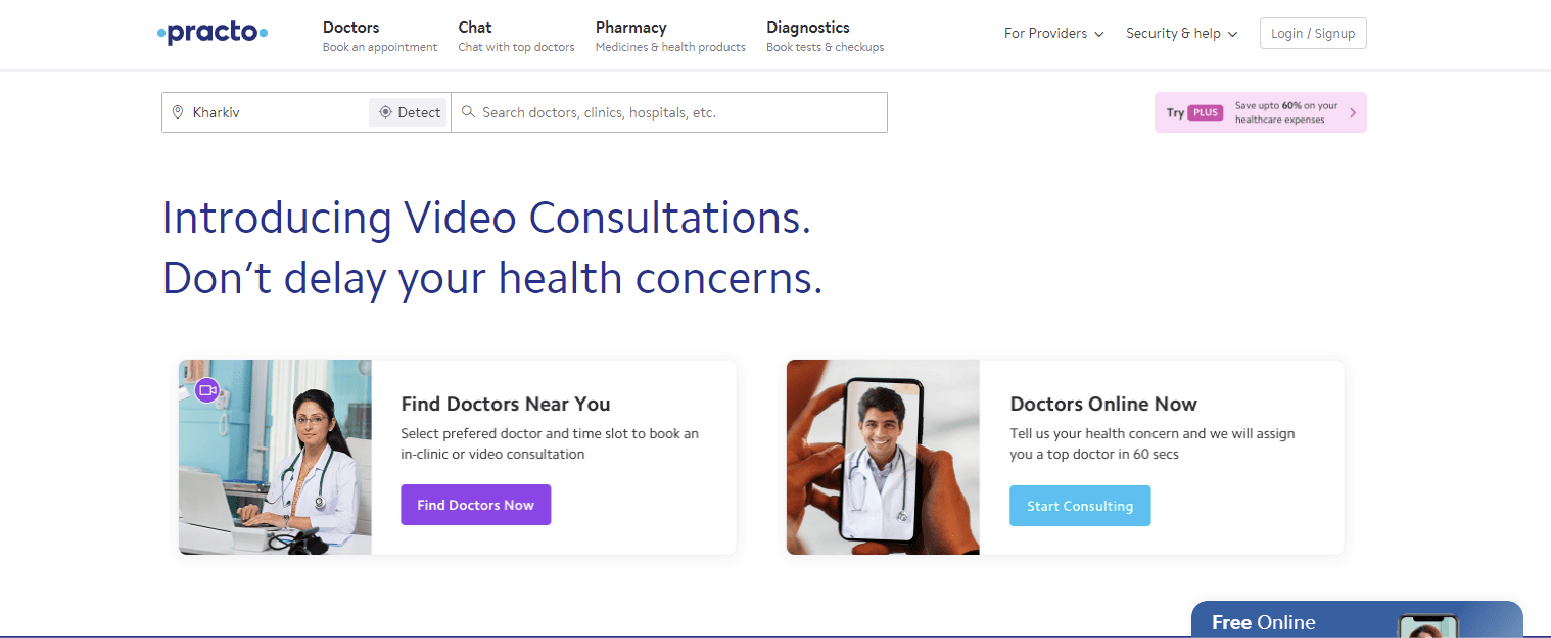A detailed and organized online platform interface is depicted, promoting comprehensive healthcare services. The screen displays the Practo app, providing features such as chatting with doctors, accessing pharmacies, diagnostic options for providers, and strong security measures. Users have the choice to log in or sign up as part of the streamlined experience. The interface highlights options such as detecting clinics, searching for doctors, and selecting hospitals, with efficient search and filter tools.

A prominent section introduces video consultations, encouraging users not to delay their health concerns and to easily find doctors nearby. Specific instructions guide users to select their preferred doctors, choose a convenient time slot, and book either an in-clinic visit or a video consultation. For immediate needs, the app offers a rapid connection to top doctors in just 60 seconds with an option to start consulting right away.

The illustration supports this functionality: on one side, a doctor is shown on the screen of a phone that a user is holding, highlighting the ease of accessing medical advice via mobile. To the left, another doctor is depicted sitting on a chair with a laptop in front of her, a stethoscope around her neck, and glasses on, in a professional setting against blue walls. At the bottom right, it indicates ‘Free Online’ services with the visible top portion of a cell phone and a faint view of someone’s head, underscoring the availability and accessibility of these services.